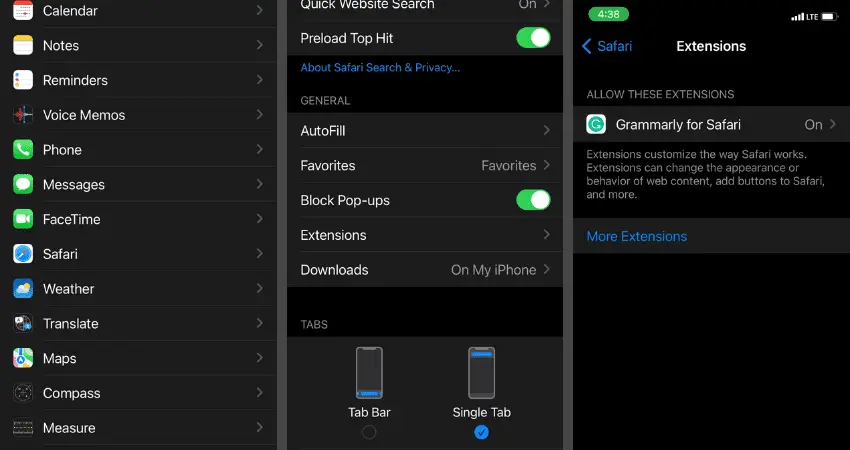### Detailed Caption for the Image

The image displays three vertical cell phone screens, all featuring interfaces with black backgrounds. 

#### First Screen:
- **Content**: This screen showcases a list of apps, each accompanied by an icon positioned to the left and white text. The apps displayed are: 
  1. Calendar
  2. Notes
  3. Reminders
  4. Voice Memos
  5. Phone
  6. Messages
  7. FaceTime
  8. Safari
  9. Weather
  10. Translate
  11. Maps
  12. Compass
  13. Measure
- **Design**: Each app is separated by thin gray lines, and a small gray arrow is placed to the right of each app name.

#### Second Screen:
- **Content**: At the top, partially cut off, it says "Quick Website Search" in white font with an arrow indicating its state. Below, it lists various Safari settings, including:
  - “Preload Top Hit” with a toggle switch that is turned on (green on the left, white circle on the right).
  - A blue font link titled "About Safari Search & Privacy".
  - **General Settings** section includes:
    - "Autofill" with an indicator.
    - "Favorites" with an indicator.
    - “Block Pop-ups” turned on (green on the left, white circle on the right).
    - "Extensions" with an indicator.
    - "Downloads" showing "My iPhone" with an indicator.
- **Tabs Section**: Two phone image options:
  - The left image is black with a blue bar at the bottom and labeled "Tab Bar" with an unchecked circle below.
  - The right image shows a blue bar at the top labeled "Single Tab" with a filled blue circle.

#### Third Screen:
- **Top**: Displays the time, "04:38", in a green horizontal oval with a white font, accompanied by a battery icon to the right.
- **Content**: 
  - The word "Safari" in blue with a left-pointing indicator on the left.
  - The word "Extensions" centered in bold white font.
  - Below, a header, "ALLOW THESE EXTENSIONS", in all caps.
  - Displays the Grammarly logo with the text "Grammarly for Safari” and a right indicator showing it is switched on.
  - An explanation detailing, "Extensions customize the way Safari works. Extensions can change the appearance or behavior of web content, add buttons to Safari, and more."
  - Finally, a blue link that reads "More Extensions."

This comprehensive caption outlines each screen's content and design specifics, offering a clear visualization of the depicted interfaces.